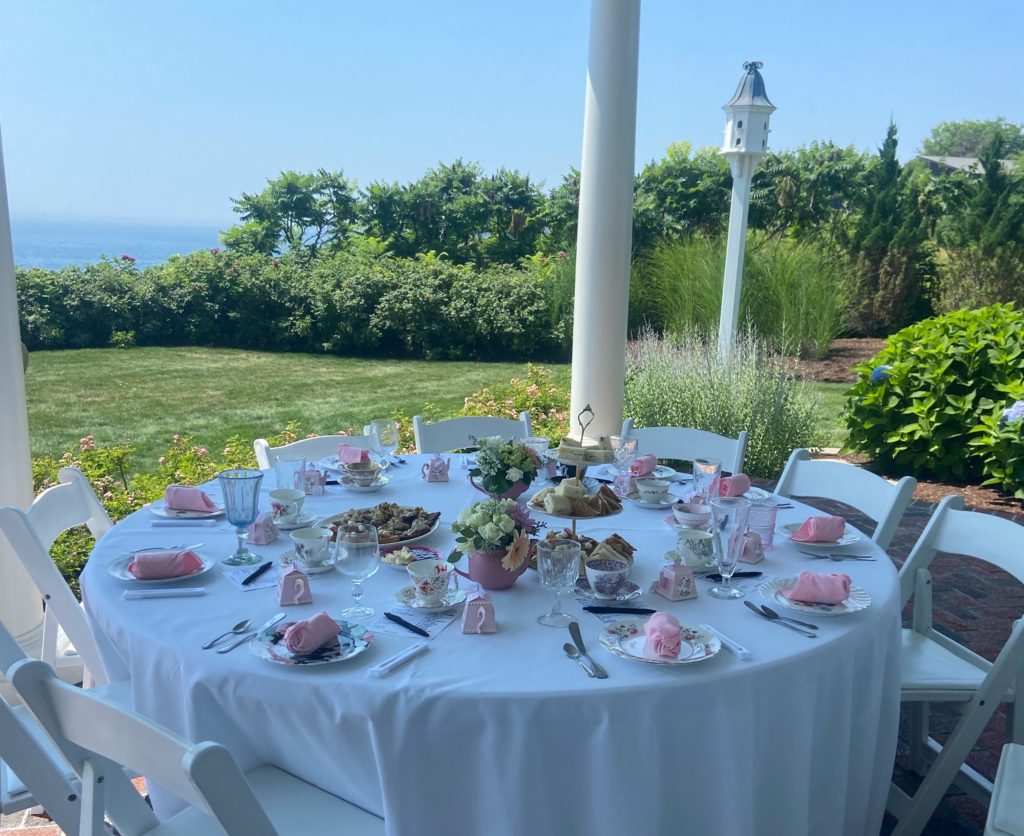This outdoor photograph captures a serene tea party set under the shade of a gazebo or overhang on a bright, sunny day. The foreground features a round table draped in a pristine white tablecloth, surrounded by elegant white chairs. Each of the approximately 11 place settings includes a decorative floral plate with a pink linen napkin neatly rolled on top, accompanied by a teaspoon and butter knife to the left. 

Floral tea cups and various types of glasses are carefully arranged around the table, hinting at a sophisticated gathering. At the center, potted plants with flowers bloom inside teacups, alongside an assortment of plates bearing delicate pastries and sandwiches cut into squares and triangles, presented on a three-tiered holder. Small gift boxes shaped like tea kettles sit at each place setting, suggesting a charming, thematic touch.

The backdrop reveals a lush garden of green leaf trees and shrubs, with a well-manicured grass lawn extending towards more greenery at the property's edge. In the distance, the serene expanse of the ocean meets the horizon, adding to the picturesque setting. The entire scene is bathed in sunlight, evoking a sense of peacefulness and elegance.